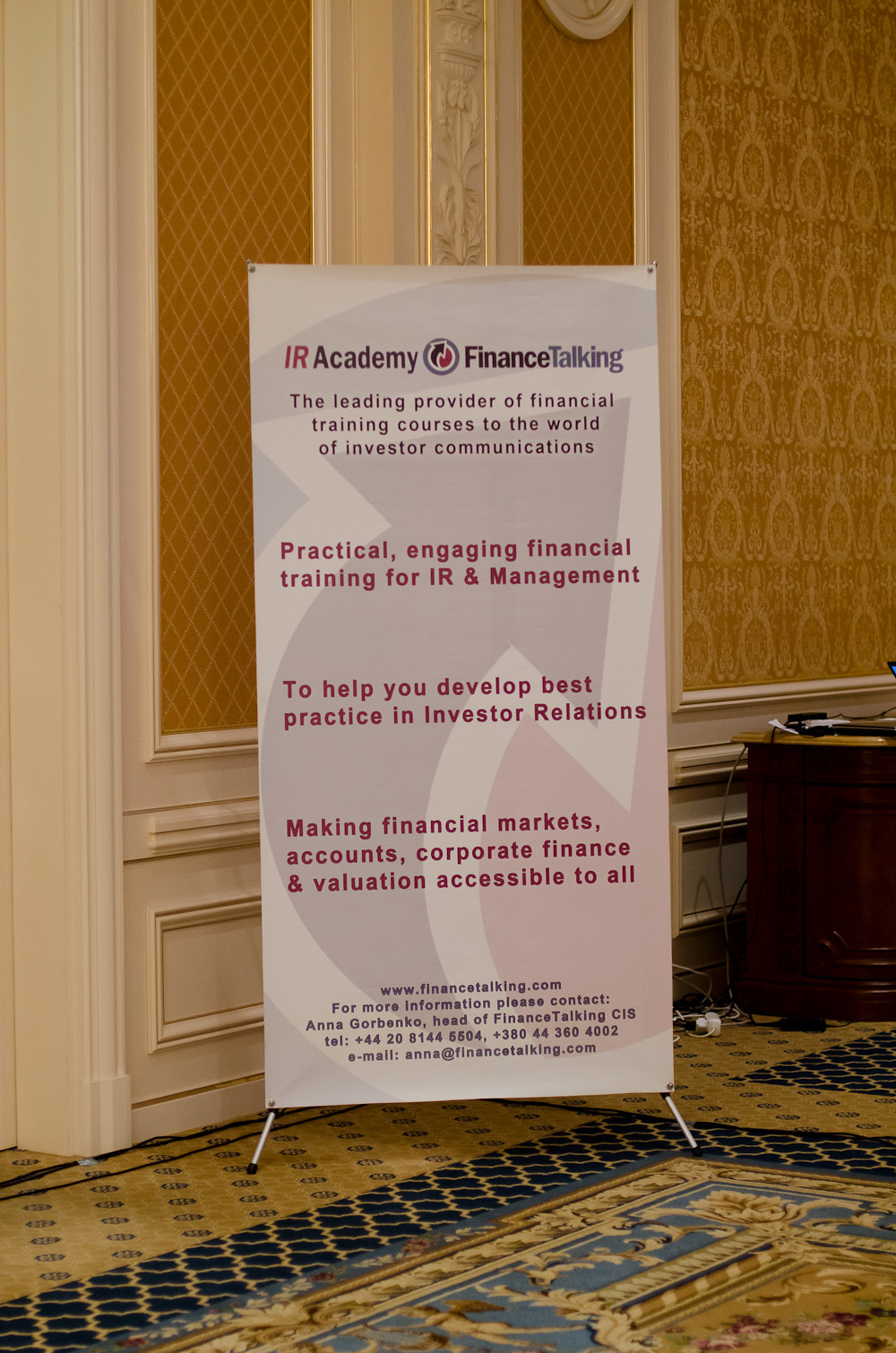The image captures the ornate interior of what appears to be a luxurious hotel or high-end event room. The floor is adorned with an elaborate carpet featuring primarily blue and gold hues, with intricate geometric shapes, flowers, and flourishes. The walls are embellished with gold-patterned wallpaper and accented by white molding, contributing to the room's opulent atmosphere.

In the foreground, a vertical rectangular sign stands on the richly decorated carpet, supported by metal legs. The sign has a white background with overlapping blue and red arrow logos that form a circular design. It prominently displays "IR Academy" and "Finance Talking," highlighting itself as the leading provider of financial training courses to the world of investor communications. Below this title, the sign details its offerings: "Practical, engaging financial training for IR and management to help you develop best practices in investor relations," followed by "making financial markets, accounts, corporate finance, and valuations accessible to all." At the bottom of the sign, in much smaller text, there's the website www.financetalking.com, contact information for Anna Gorbenko, Head of Finance Talking CIS, along with her telephone numbers and email address.

To the right of the sign is a vintage, dark brown wooden desk with a golden-yellow top. Various items, including laptops, wires, chargers, and papers, are scattered atop the desk, with some cables trailing down to the floor. The room’s overall lavish décor, combined with the detailed sign, creates an impression of a sophisticated setting focused on high-level financial training.